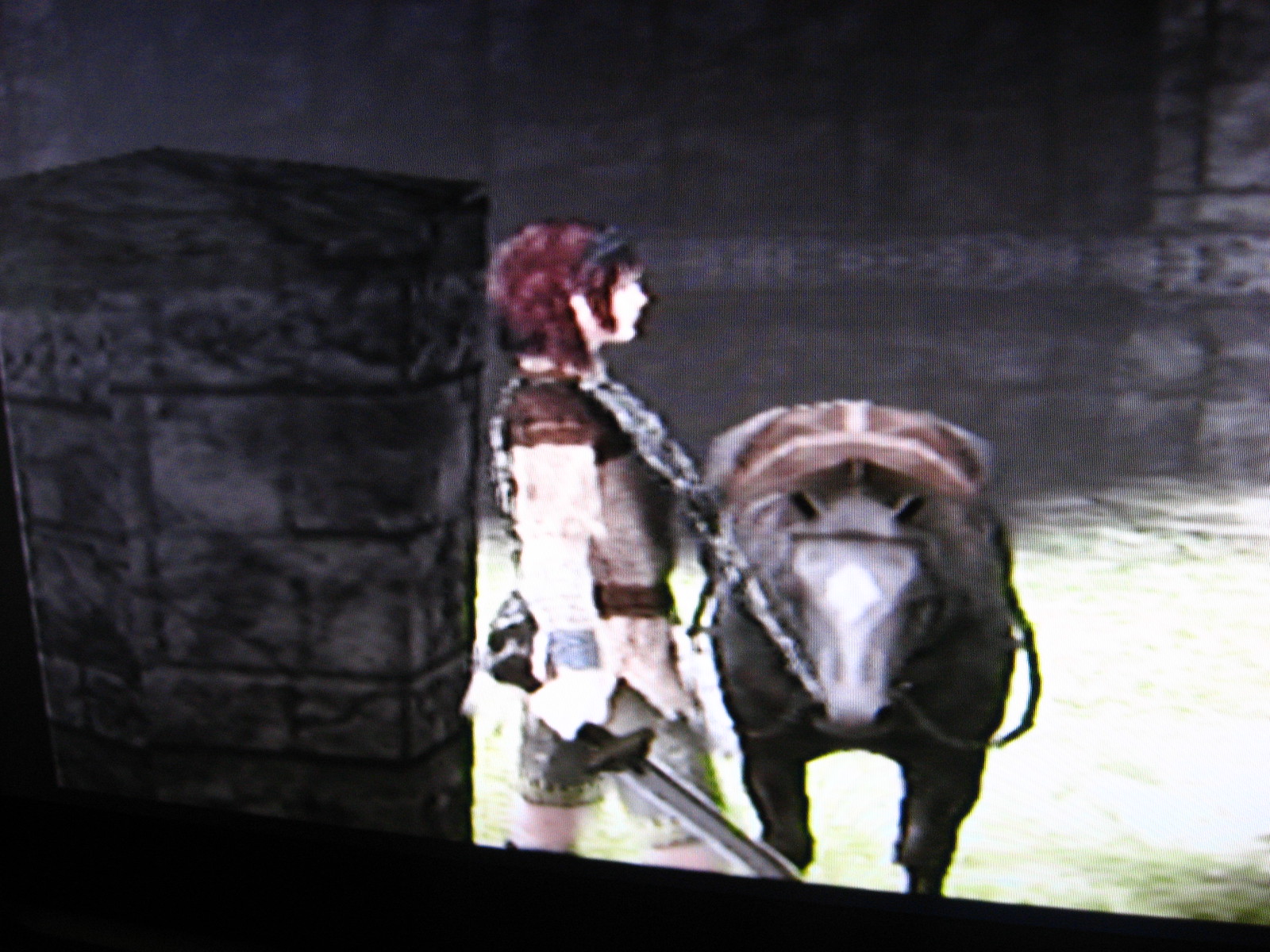This image is a screenshot from an early to mid-2000s video game, characterized by its blocky, less finely rendered graphics reminiscent of classic titles like Resident Evil 2 or 3. It depicts a woman standing in the courtyard of a stone building, with lush green grass underfoot. She faces towards the right, dressed in a brown, medieval-style outfit that may include armor, though the details are not entirely clear. Wielding a sword in her right hand, she has short, reddish-brown hair reaching her shoulders at the back. Next to her stands a grayish-brown horse, which is directly facing the camera. Prominently, the left third of the image is obscured by a large stone pillar in the foreground.